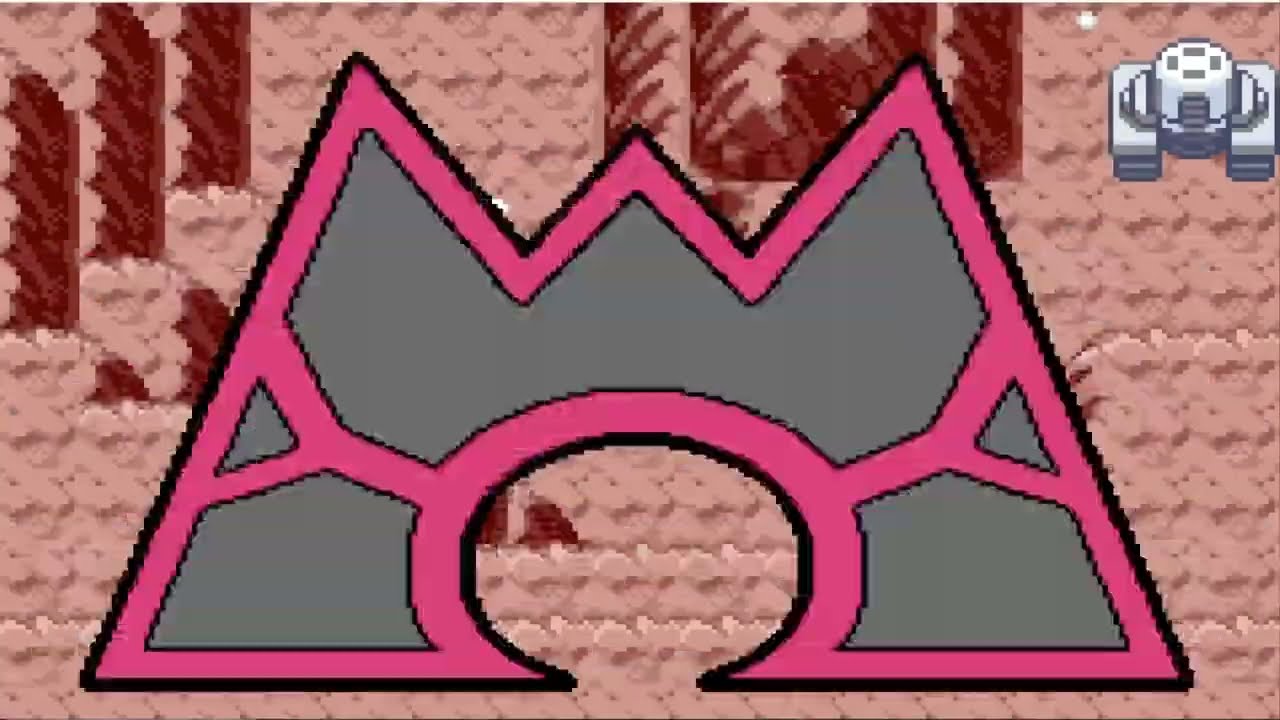The image is a pixelated, top-down view, likely from a video game with a desert-style, tiled pattern ground. Prominently in the center is a stylized design resembling an upside-down letter M or a W, with sharp, pointed tips. The structure has two arms diverging downward, forming a base with a semi-circle cut out, exposing the beige and pink backdrop with vertical light brown or dark brown strips. The central design features bright pink outlines and a gray filling. This M-shaped or crown-shaped figure appears to represent a person or a robot wearing headphones. Additionally, in the upper right corner, there is a digital white and gray army tank or generator, adding to the intricate details of the scene.